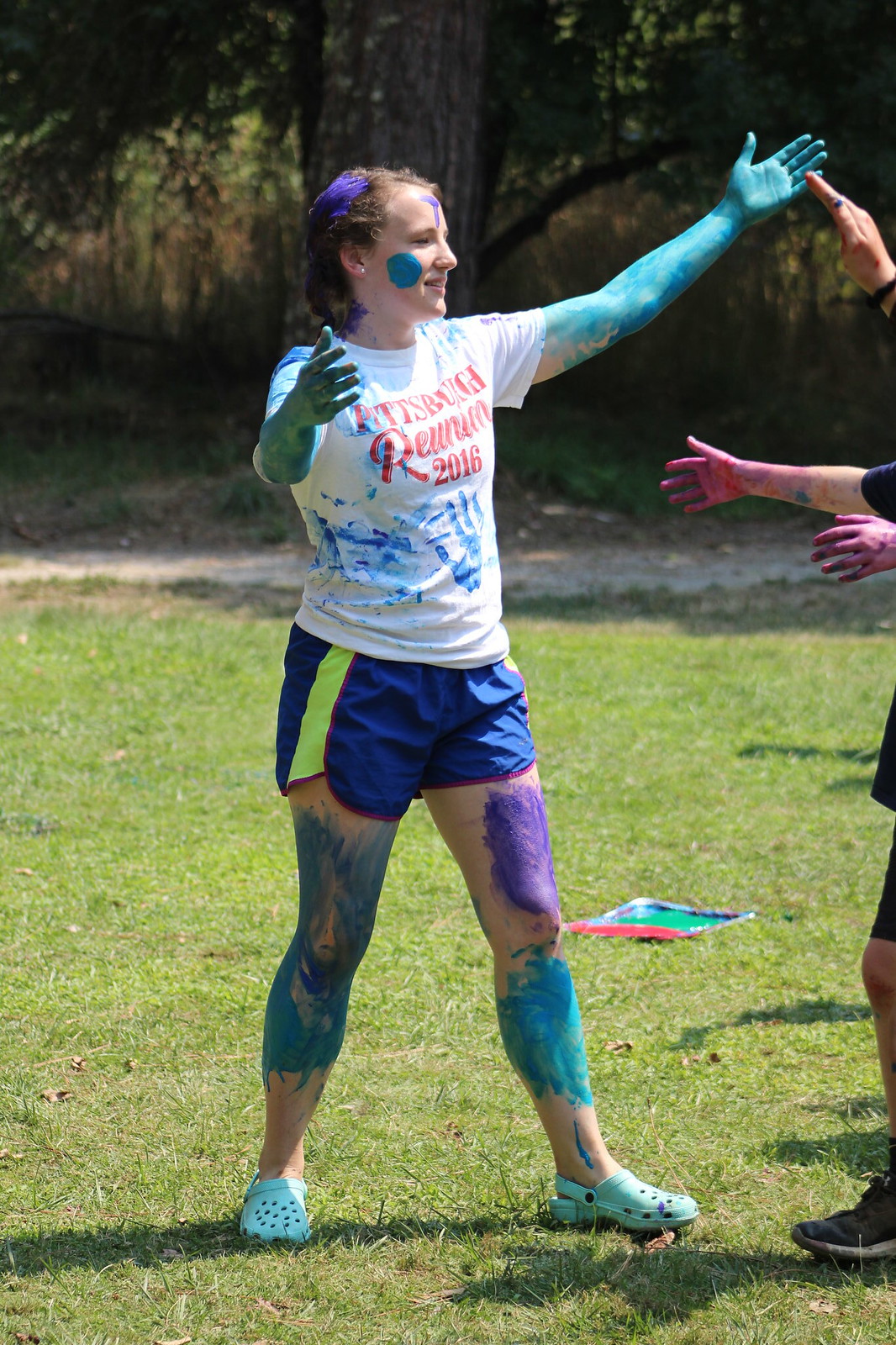In this vibrant, vertically aligned photograph, a woman stands at the center of a grassy area, her white t-shirt emblazoned with "Pittsburgh Reunion 2016" in red. She is covered in an array of paint colors: her left forearm and palm are painted green, purple paint streaks through her hair, and blue splotches adorn her face. Her turquoise Crocs match the blue and turquoise paint splattered across her thighs and shins. 

The scene unfolds outdoors in the middle of the day, likely during a group event or playful activity, as suggested by the colorful sheets of painted paper lying on the ground around her. The background is slightly blurred but identifiable as a wooded area with green trees and a dirt path cutting across the image. 

The woman stands with her arms outstretched as though inviting a hug or participating in a playful interaction, facing another individual partially visible in the frame who wears a black shirt, black shorts, and black tennis shoes. Additional painted arms reach toward her, emphasizing the communal and joyous nature of the event depicted in the image.